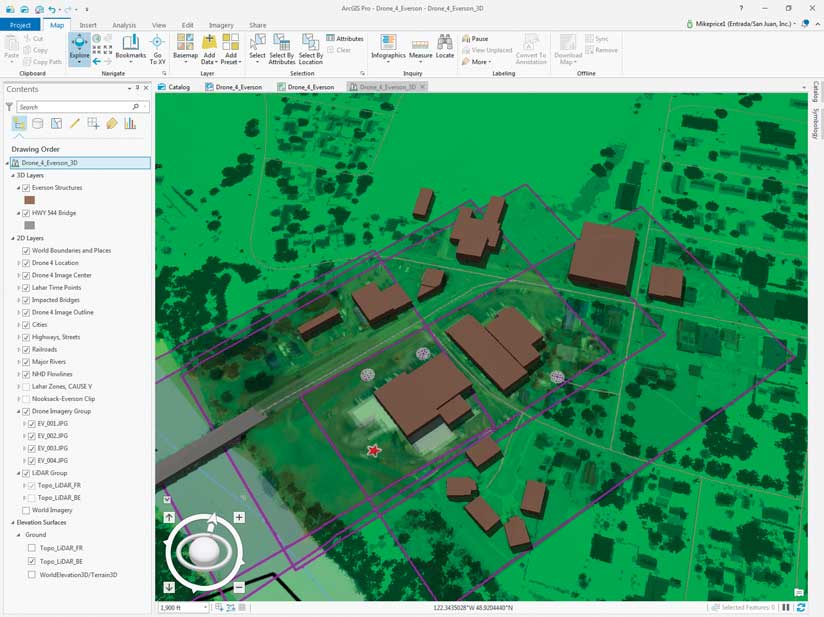The image displays a screenshot of a computer program, which appears to be a city planning or architectural software. The main interface reveals a green map layout of a small town section, possibly the entire town, presented in a grid format from a bird's-eye view. The map features simplistic brown squares representing building blocks, likely warehouses or similar structures, devoid of intricate details. These buildings are set against a backdrop of green ground and are interspersed with roads and areas of darker green representing greenery.

On the left side of the screen, there is a toolbar labeled "Contents" with a search bar and a list of items, many of which have checkboxes that are checked off. At the top, a ribbon menu includes various options such as "Project," "Map," "Insert," "Analysis," "View," "Edit," "Imagery," and "Share," along with specific map-related options like "Explore," "Bookmarks," and "Add Data." The bottom left corner includes navigation keys similar to those found in Google Maps, used to manipulate the map view. The overall layout of the program resembles that of typical Windows software applications, with toggleable and clickable lists and checkboxes on the left, and multiple options in the top bar.